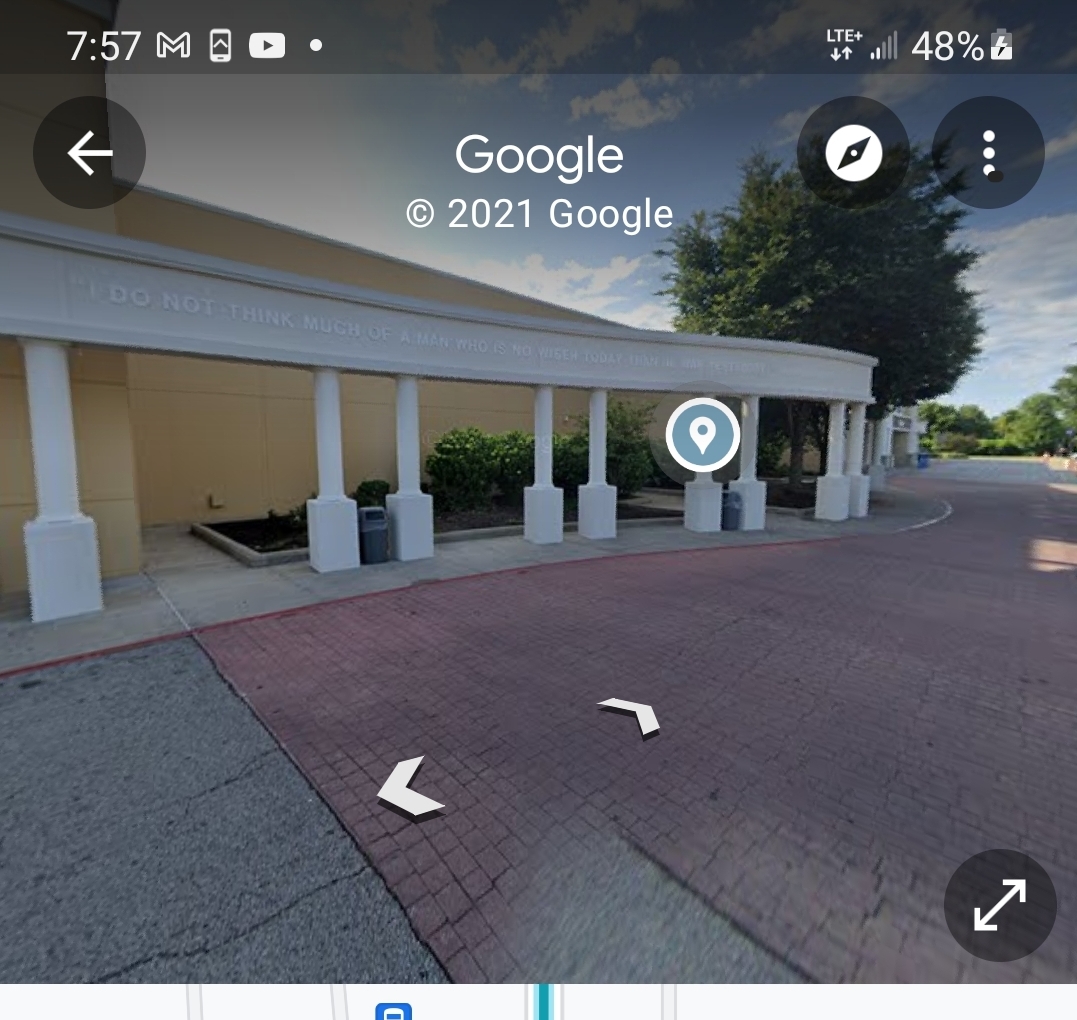The image displays a Google Street View map focusing on the front of a shopping center, captured in 2021. The phone's battery level is at 48%. The scene includes an asphalt roadway interspersed with a pattern resembling paving stones. A yellow building dominates the view, featuring a colonnade with columns approximately every 10 feet. Each column has a square base, with trash cans positioned between every other pair. The colonnade stretches into the distance, but no doorways are visible. The parking lot includes patches of greenery, with trees dotting the landscape intermittently.